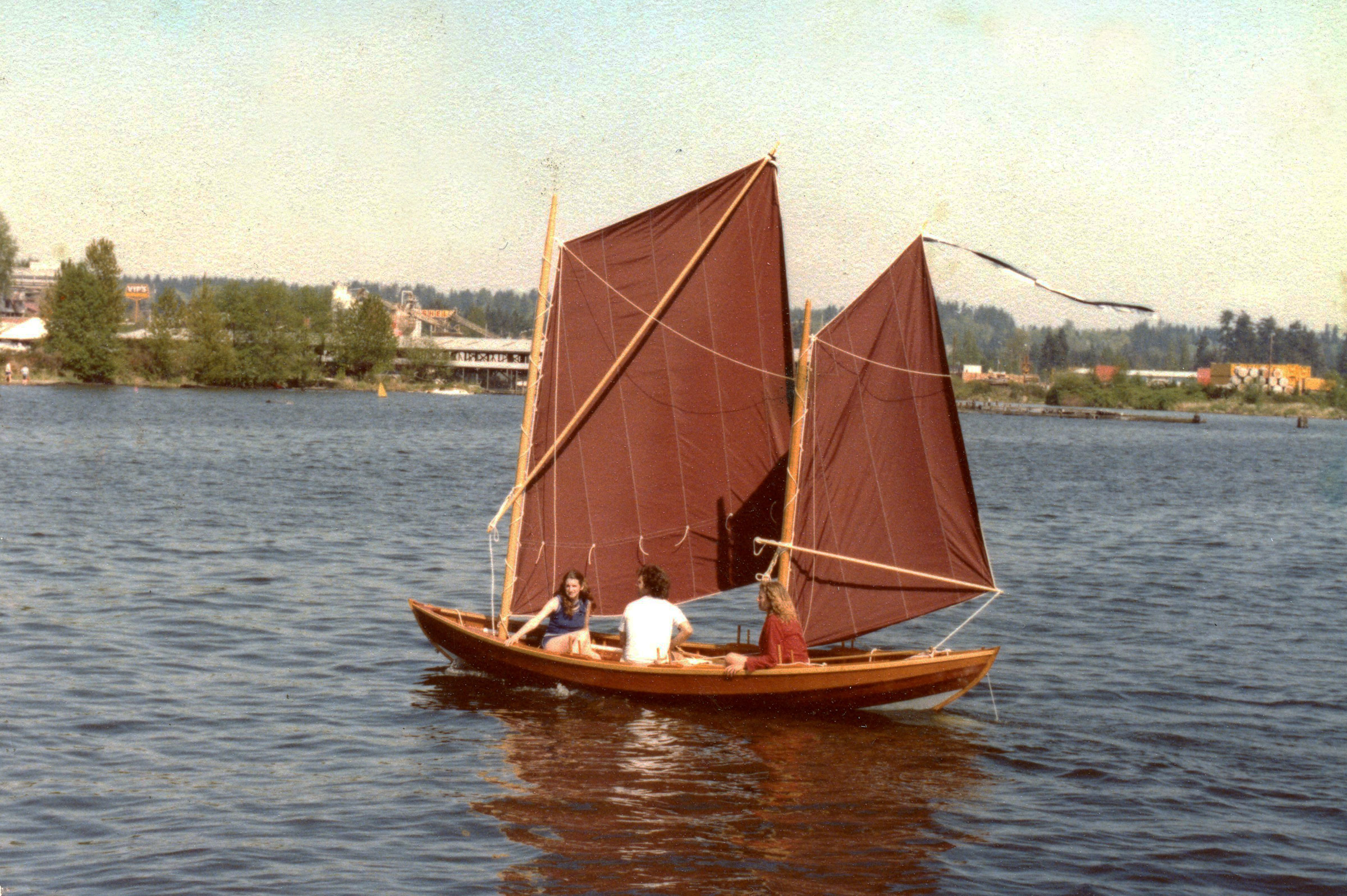This color photograph, which appears somewhat faded and degraded over time, seemingly dates back to the 1970s. It depicts a tranquil scene of a small wooden sailboat in the middle of a large, mostly still, dark blue lake or river. The boat, which resembles a canoe but with two brown sails, is crafted from wood and has a brown base. It carries three people: a woman in a blue sleeveless shirt at one end, a man in a white short sleeve shirt in the middle, and another woman in a red long sleeve top at the other end. The smaller sail is adorned with a ribbon at the top. In the background, trees and buildings line the water’s edge, with the sky above appearing primarily light yellow, likely due to color fading, with only patches of blue visible. The overall scene suggests a peaceful day underscored by the clear sky and gentle ripples on the water.